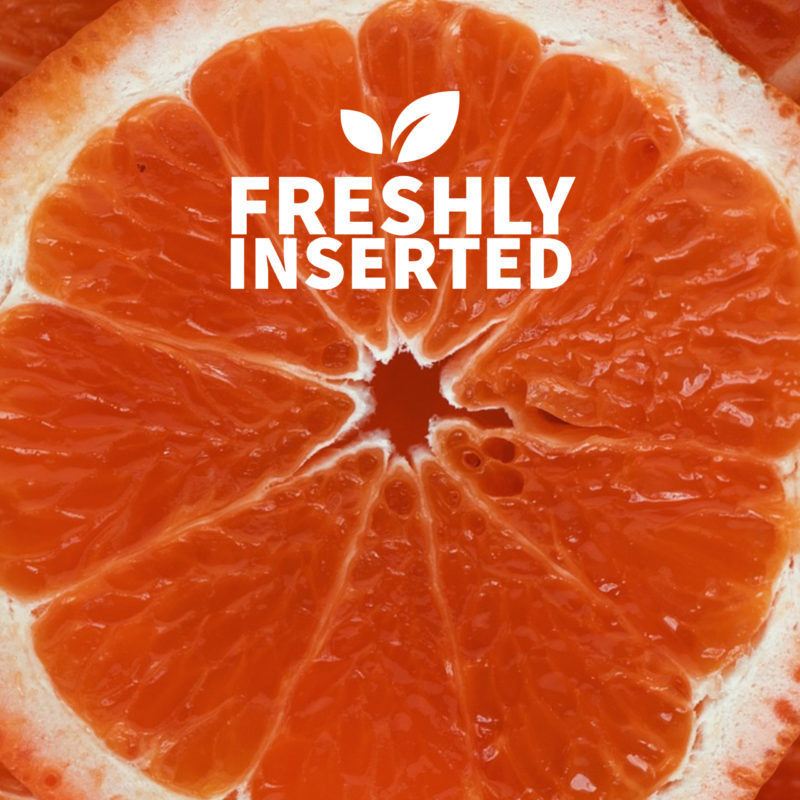This vibrant, square close-up photograph showcases a freshly sliced ruby red grapefruit, capturing its intricate details and colors vividly. The image sharply zooms in on the circular cross-section of the fruit, revealing its segmented, triangular flesh in hues ranging from pinkish-red to deep orange, surrounded by a conspicuous white rind. The skin at the edges displays a blend of orange, reddish, and brown tones. The composition is bright and clear, accentuated by natural light that enhances the fruit's texture and color. Overlaying the top center of the image, white sans-serif text reads "freshly inserted," accompanied by a minimalist icon of two leaves, with the larger leaf on the right. The overall clarity and brightness make this a striking, easily readable image.